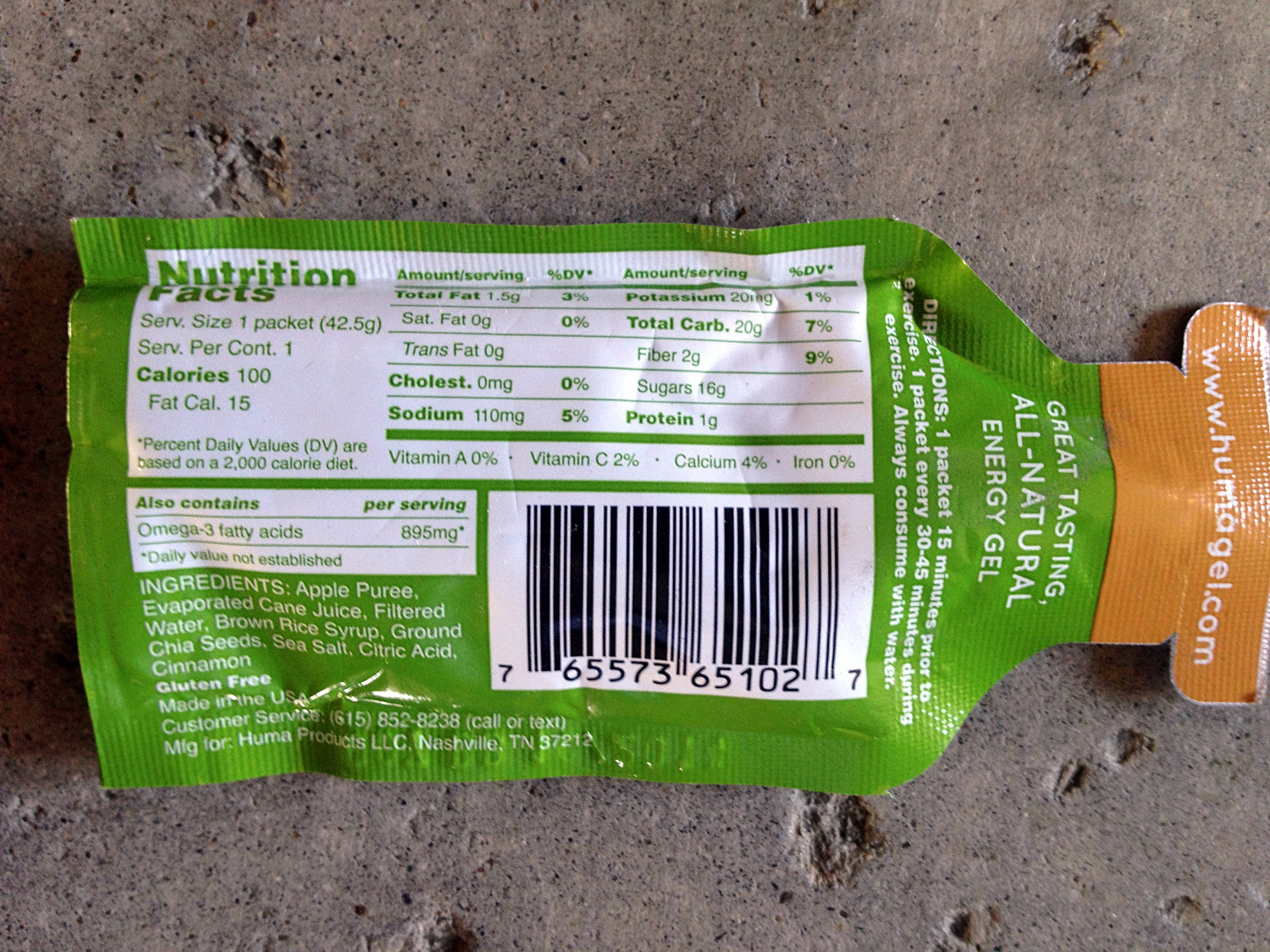This photograph features an energy gel packet resting on a marbled cement floor, characterized by darker, blacker holes and scattered black spots. The packet is viewed from above, lying sideways with its bottom facing left and top facing right. The green body of the pouch contrasts with its orange top, which prominently displays the website "www.humagel.com" in white text. Just below this, the packet also advertises "Great Taste, All-Natural Energy Gel." The backside of the pouch includes a white nutrition facts box, a barcode, and an ingredients list. Key ingredients mentioned are apple puree, evaporated cane juice, and brown rice syrup, and it also contains omega-3 fatty acids. The serving size indicated is one packet.